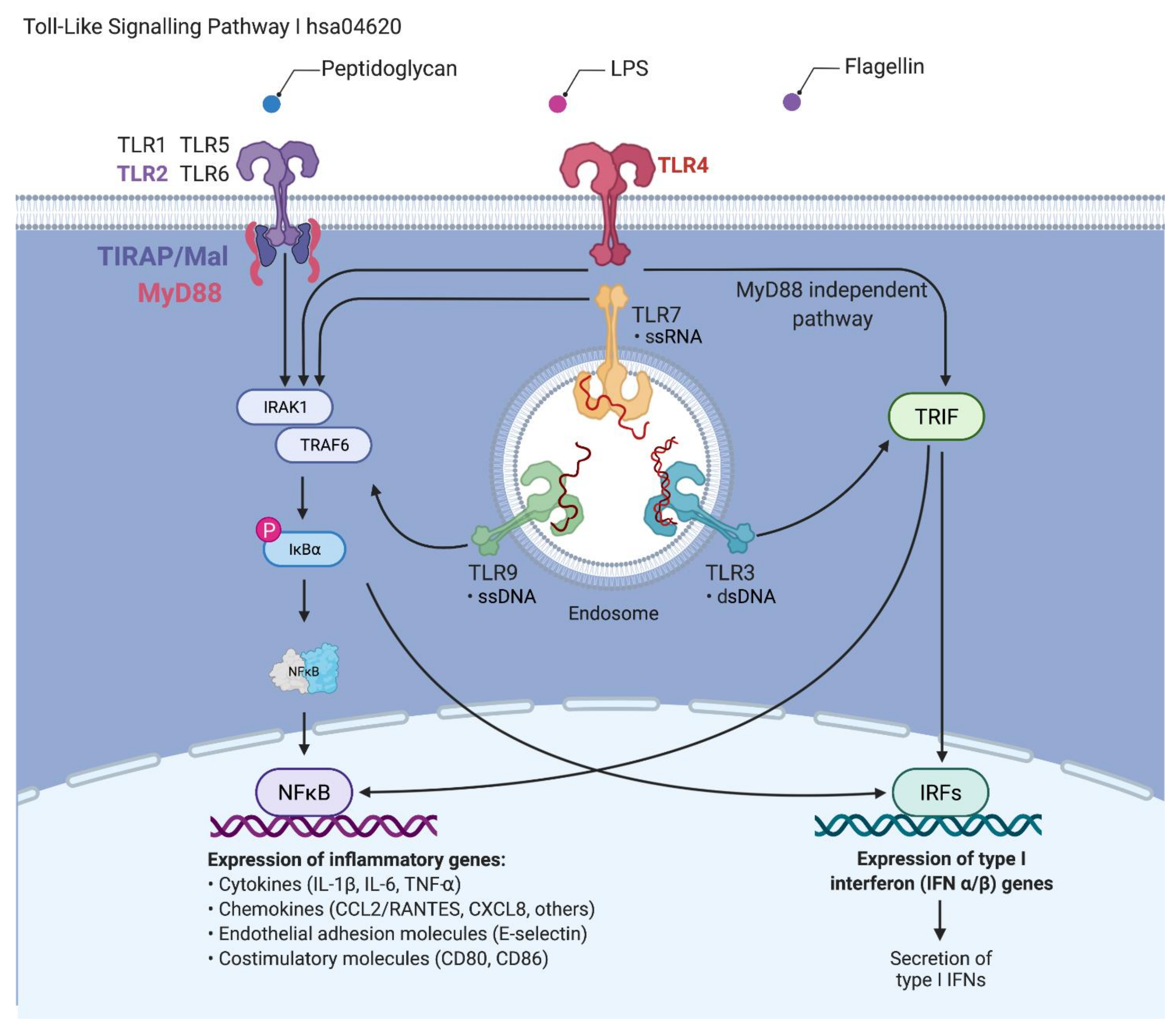This diagram, labeled "Toll-Like Signaling Pathway HSA 04620" at the top, intricately maps out the complex interactions within a cell related to gene expression. The topmost section features callouts for peptidoglycan, LPS, and flagellin. These elements appear to interact with various Toll-Like Receptors (TLRs), specifically TLR1, TLR2, TLR5, and TLR6, suggested by their recurring labels. In the center of the diagram is a white circle containing three anchor-like shapes in green, orange-yellow, and blue, labeled TLR7 (ssRNA), TLR9 (ssDNA), and TLR3 (dsDNA) respectively. Surrounding this central circle, numerous arrows point towards and away from an array of labeled components such as IRAK1, TRAF6, and TIRAP-MAL-MI-D88, indicating complex signaling processes. Lower sections of the diagram delve into gene expression details, with left-side annotations noting the expression of inflammatory genes, cytokines, chemokines, endothelial adhesion molecules, and co-stimulatory molecules. On the right side, it emphasizes the expression of type 1 interferon (IFN) genes and their secretion pathways, marked by blue squiggles and the label IRFs. Altogether, the diagram densely showcases the myriad interactions and pathways involved in cellular signaling and gene expression, although much of it remains highly technical and specialized.